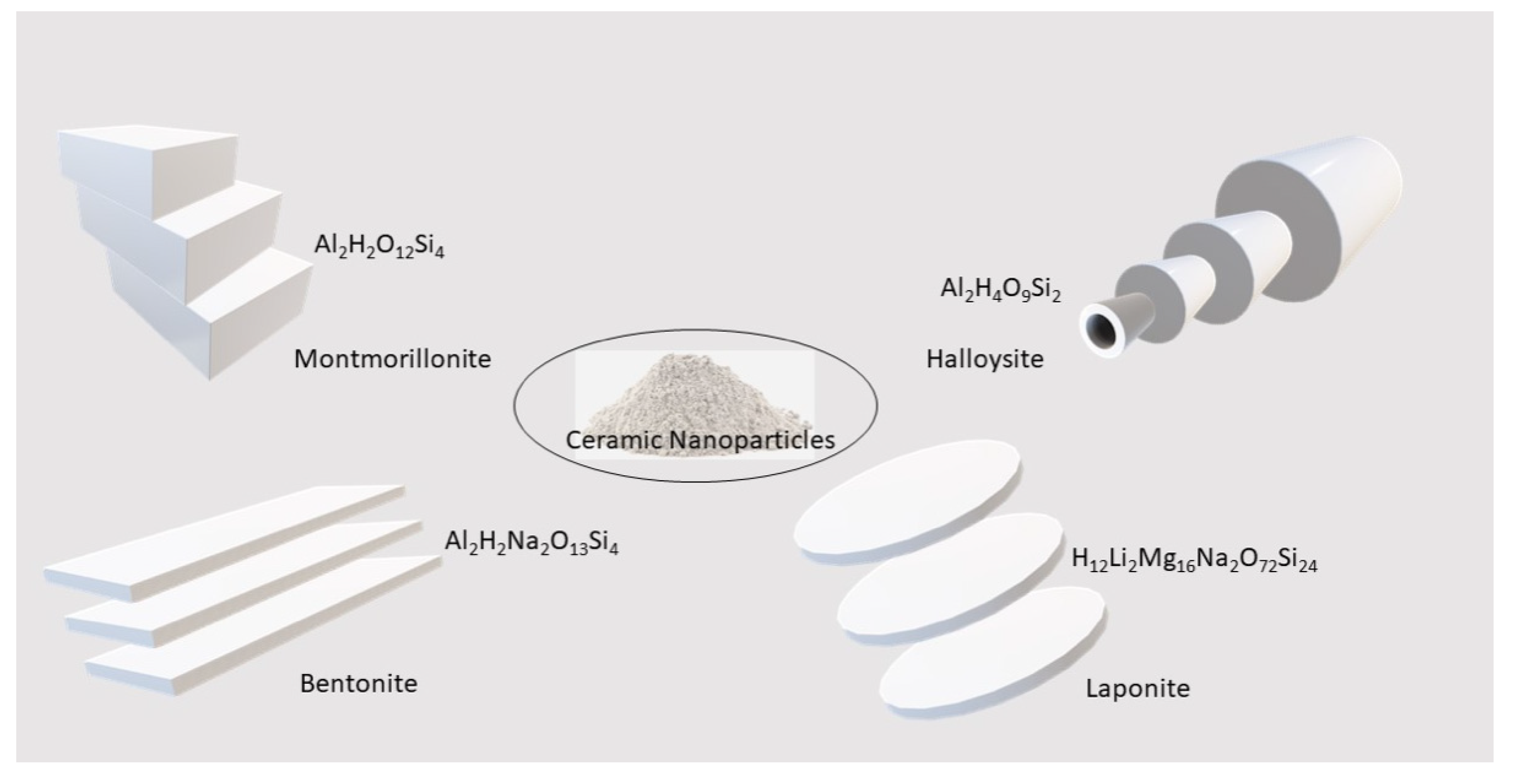This detailed scientific diagram displays four different mineral compounds, each represented by a three-dimensional object with its chemical formula and common name. In the center, encircled by a black oval, lies a small mound of gray powder labeled as ceramic nanoparticles. In the upper left corner, three white rectangular blocks are stacked in a staircase formation, marked with the chemical formula Al₂H₂O₁₂Si₄ and labeled Montmorillonite. The top right corner features white and gray conical shapes similar to a tilted vase, identified as Halloysite with the formula Al₂H₄O₉Si₂. At the bottom left, three flat sheets of white material form a staircase-like structure, corresponding to Bentonite, characterized by the chemical composition Al₂H₂Na₂O₁₃Si₄. Finally, the lower right corner presents three thin, white circular disks representing Laponite, defined by the formula H₁₂Li₂Mg₁₆Na₂O₇₂Si₂₄. The overall aesthetic resembles a slide from a scientific presentation, utilizing cream and white colors with black text for contrast, and detailed shadows to emphasize the three-dimensional geometry of each object.